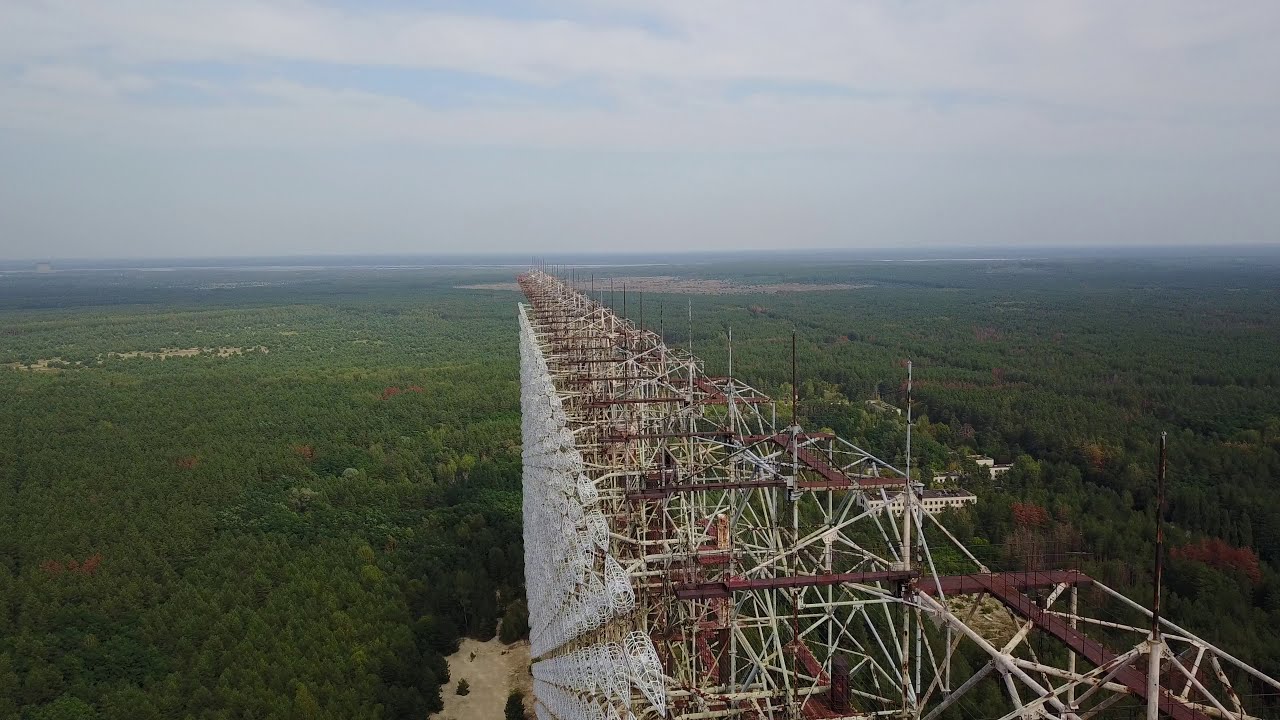The image is a color photograph taken from a high vantage point, likely by a drone, in landscape orientation. It captures a large, narrow, and very tall bridge-like structure under construction, made from a network of intersecting white bars and rust-colored horizontal beams and walkways. The structure is situated in a rural area, surrounded by dense woodland that stretches to the horizon, with patches of brown dirt visible in some clearings. A significant white building can be seen on the left side of the image. The sky above is a light blue with a mix of white and light gray clouds. The photograph uses a realistic and representational style.